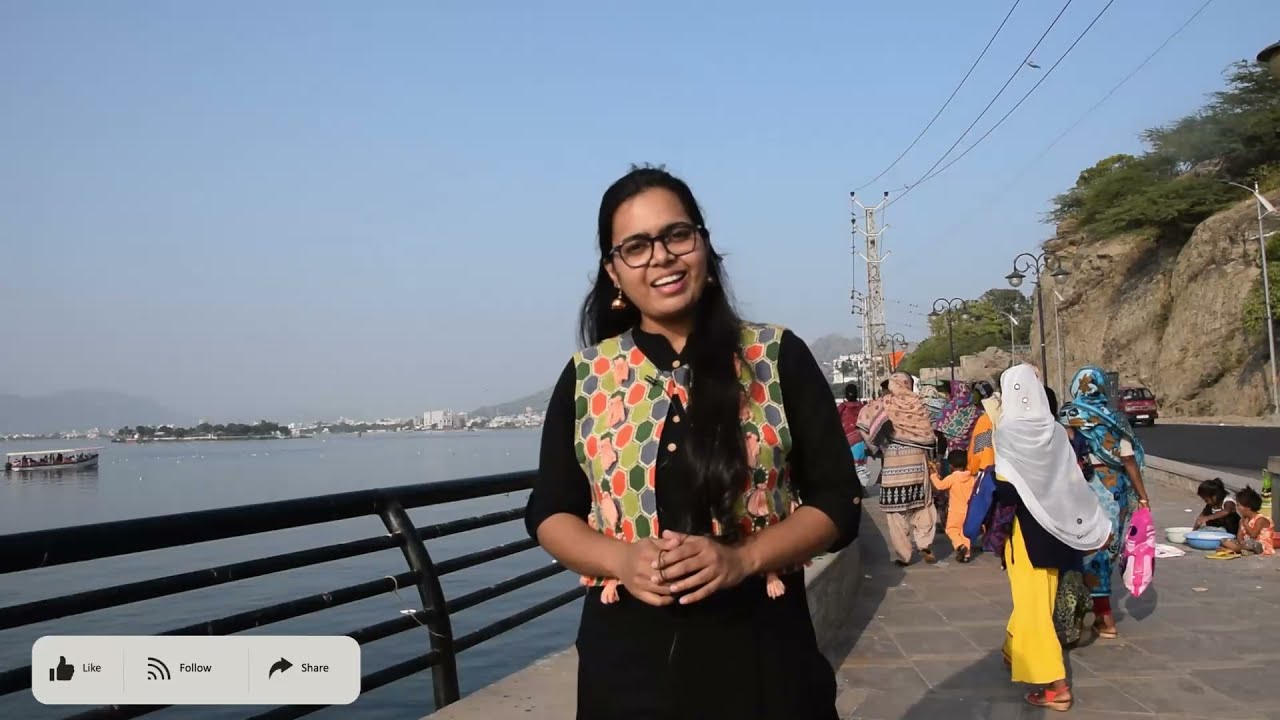The image captures a woman standing on a cement walkway beside a large body of water, which could be an ocean or a lake, framed by a black horizontal railing. She has a tanned skin complexion, wears black glasses and long black hair cascading over her shoulders. She's dressed in a solid black outfit adorned with a vest featuring large, vibrant circular patterns in blue, green, orange, and pink. Behind her, you can see a diverse landscape with a boat on the water, mountains, a cityscape in the far distance, and a clear blue sky. To her right, a road runs parallel to the water, where a vehicle can be seen traveling. Nearby, two children appear to be playing with bowls, and several people, dressed in dark clothes and head wraps, are walking away from the camera, seemingly unaware of the woman in the foreground. There are rocks and green shrubbery along a concrete cliff also visible to the right, along with power lines stretching across the scene. The image is likely a social media post, indicated by the "like," "follow," and "share" text in the bottom left-hand corner. The overall setting is serene and bathed in natural daylight.